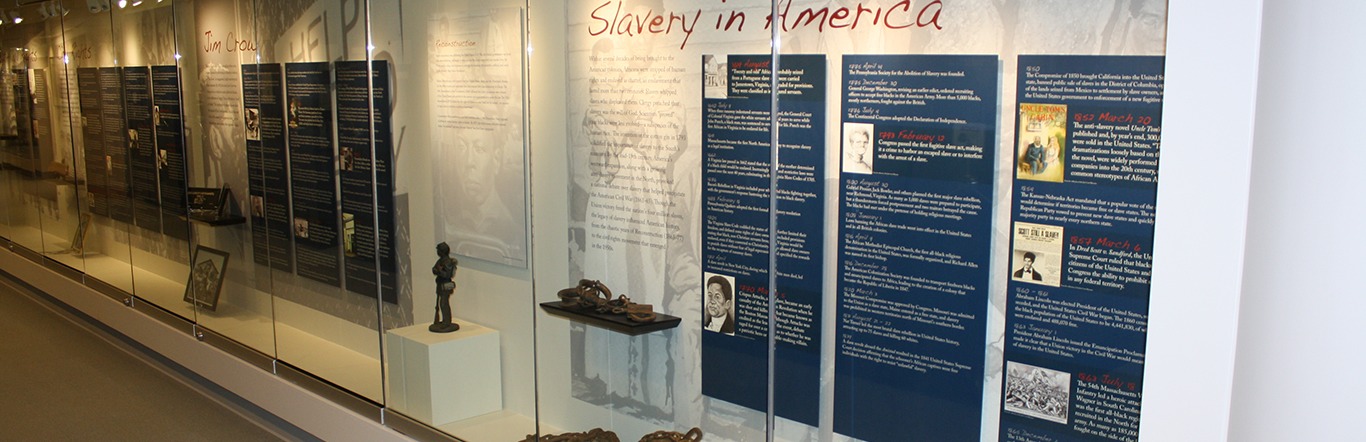In this well-lit museum exhibit focused on the history of slavery in America, various artifacts, statues, and photos are displayed behind sealed glass coverings atop secure platforms with a brown floor. Large blue posters with detailed information, such as headings like "Jim Crow" and "Slavery in America," are prominently featured behind the glass displays. The museum ensures the safety and preservation of these historical items with locked and illuminated glass cabinets, allowing visitors to engage with the comprehensive and educational content about the different aspects and eras of slavery in America.